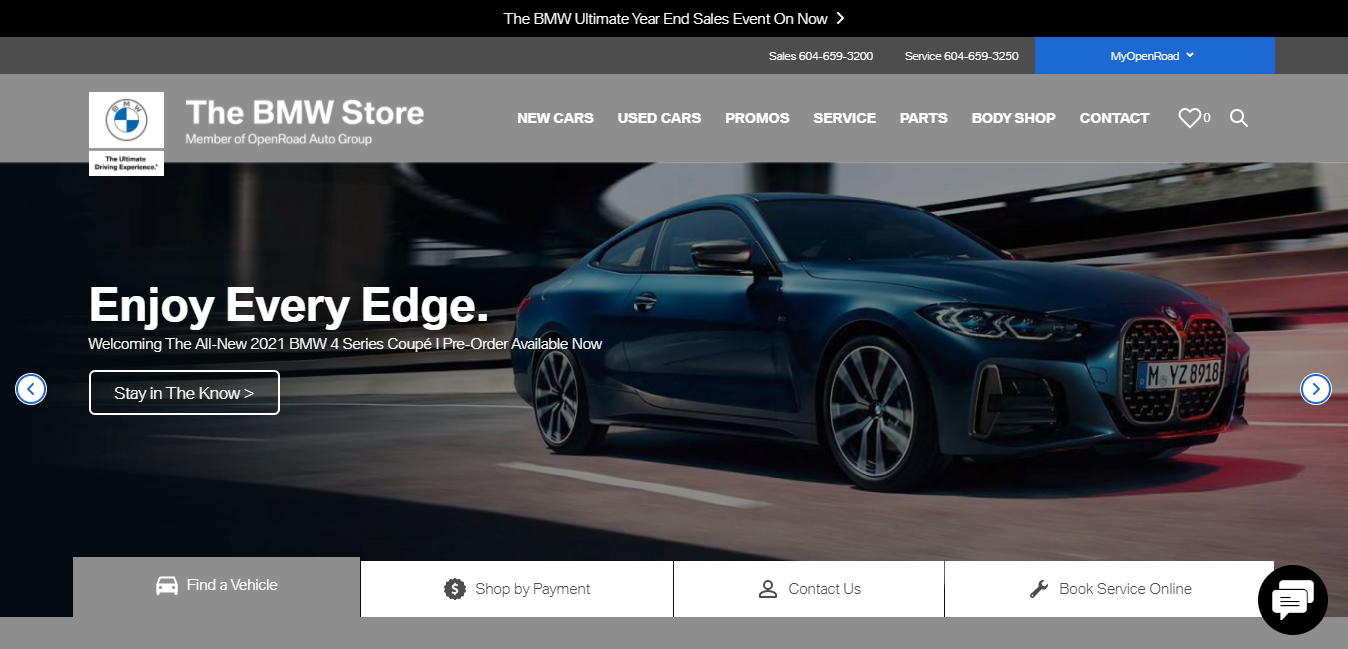The image displays a web page from the "BMW Store" featuring a promotional banner at the top. The banner, set against a black background, announces the "BMW Ultimate Year-End Sales Event" currently underway. Two categories are presented, with a blue background section to the right labeled "My Open Road". Below this, the page transitions to a gray background on the left, prominently displaying the "BMW Store". Adjacent to the store name are seven categories: New Cars, Used Cars, Promos, Service, Parts, Body Shop, and Contact, accompanied by heart and search bar icons.

Further down, there is an attention-grabbing visual of a dark blue BMW presented from both side and front angles, highlighting its silver rims and tinted front windshield. To the left of the car, in white text, is the slogan "Enjoy Every Edge". Below, another tagline reads "Stay in the Now" with a creative twist as "NWKNOW".

Toward the bottom, four options are presented. The leftmost option, in gray, is labeled "Find a Vehicle". The remaining three options, set against a white background, are "Shop by Payment," "Contact Us," and "Book Service Online." In the bottom right corner, a black circle features two white message icons, emphasizing the communication tools available.